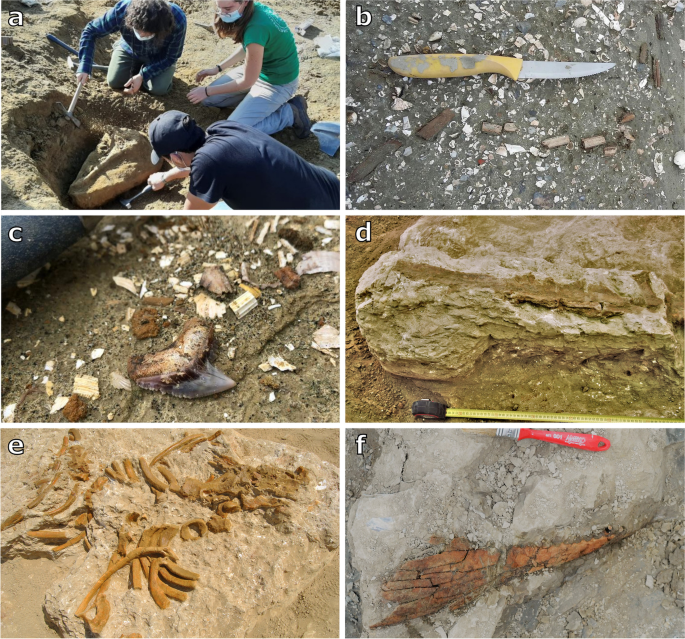This image is comprised of six individual photographs labeled from A to F, showcasing various scenes from an archaeological dig site. In photo A, located in the upper left corner, three masked students are carefully excavating what appears to be a large bone, potentially a dinosaur skull, using brushes. Photo B, situated in the upper right, displays a modern knife amidst the dirt. Adjacent to it, photo C features additional fossils surrounded by soil. Photo D highlights the excavation area on a hill with visible markings showing where work has been done. In photo E, more skeletal remains are visible, meticulously being uncovered. Lastly, photo F contains further fossils in various states of excavation. Throughout the series, measuring tapes and other tools are evident, indicating the systematic approach to the dig. The repeated depiction of bones and fossils suggests significant finds that could include both animal remains and ancient human artifacts.